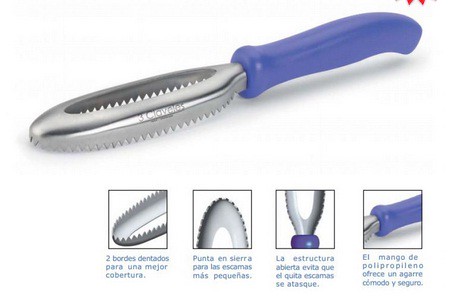The image features a kitchen implement with an iris blue plastic handle and a steel blade. This utensil has an oval-shaped tip with serrated edges on both sides, indicating it is designed for cutting. One end is flat, while the other end is equipped with these serrated teeth, which wrap around the front due to a cutout in the center. The main portion of the image displays the utensil in its entirety, while the lower half contains four close-up, annotated images that highlight specific features of the item. The annotations are in Spanish; one of them reads "Bordes dentados para un mayor cobertura," translating to "serrated edges for better coverage." These annotations provide insights into the practical use and advantages of the implement.